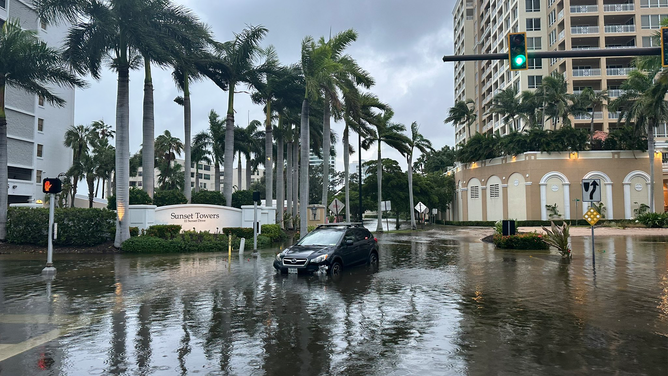In the photograph, a flooded street stretches ahead, flanked by palm trees swaying in the wind against a backdrop of dark, overcast skies. A black car is stranded mid-road, with water rising halfway up its tires. The scene unfolds before a series of high-rise buildings, including a prominent beige structure named "Sunset Towers," which sports distinctive arches and vents at its base. Traffic lights are still operational, displaying a green signal for vehicles and a red hand for pedestrians at a nearby crosswalk. The rainy weather has left the street submerged in water, though not deep enough to fully engulf the car. Scattered greenery punctuates the scene, adding a touch of nature to the urban landscape. The overall atmosphere is one of a recent storm's aftermath, with grey clouds lingering in the sky and the sense of a city temporarily brought to a standstill by flooding.